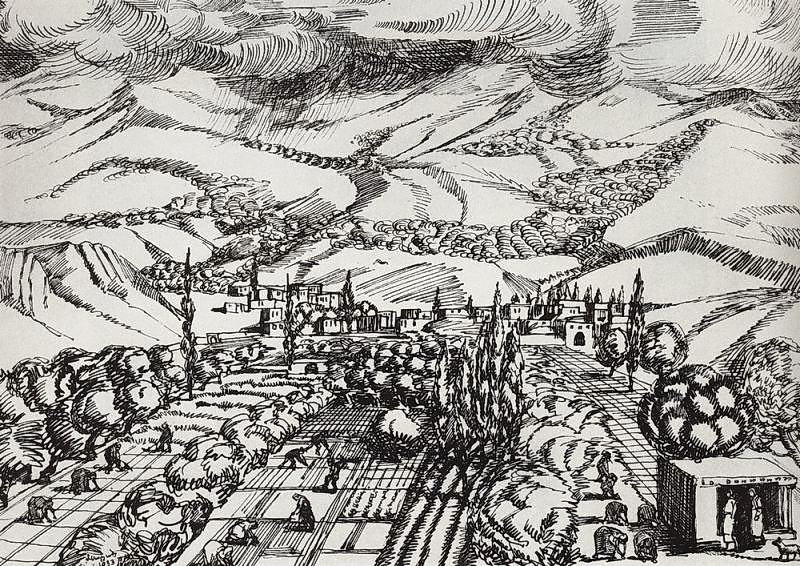This black and white drawing, reminiscent of a pencil or charcoal sketch and possibly drawn with black ink, depicts an Armenian village in a detailed and expressionistic style. Created by Martiros Sarian in 1933, the scene centers around a serene yet industrious village landscape. In the foreground, numerous figures are diligently working in the fields—harvesting, planting, and raking—suggesting a thriving agricultural community. The village itself is composed of quaint, one-story buildings, accompanied by tall, narrow trees typical of the region. Notable in the bottom right corner is a small hut with two people resting outside, accompanied by a dog. The middle ground reveals more village structures within a grid-like arrangement of roads and pathways. The background features rolling hillsides interspersed with rocks and small cliffs, eventually blending into distant mountainous ranges, adding depth and a sense of elevation to the composition. Titled "Armenian Village," the artwork captures both the essence of rural life and the rugged beauty of the surrounding landscape.